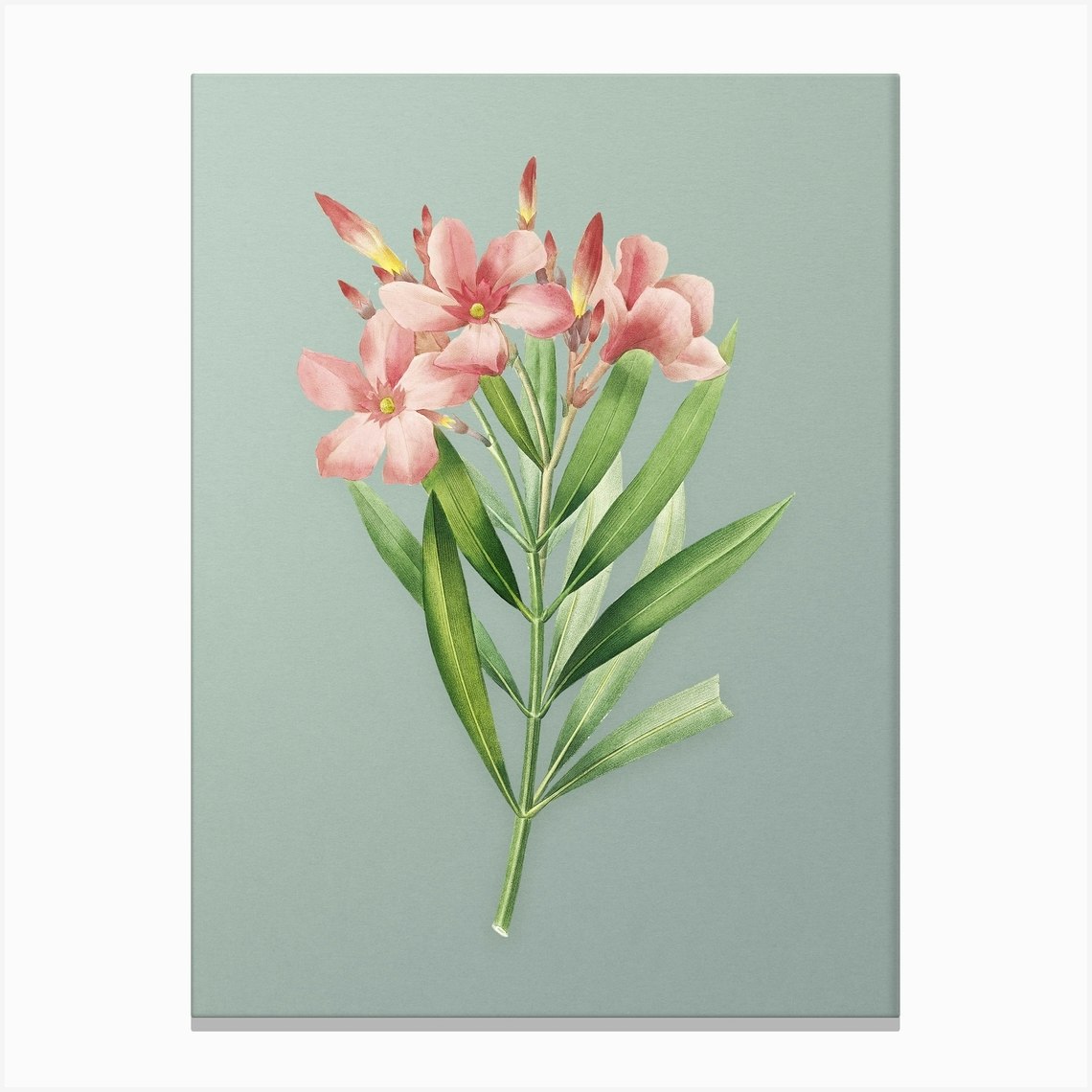This detailed caption aims to synthesize the information provided, emphasizing shared details and repeating elements:

This photograph depicts a beautifully detailed painting of a single green stem adorned with a cluster of long, narrow, and multi-toned leaves arranged in five distinct sections. Ascending the stem, the leaves lead to vibrant pink flowers, each with five petals elegantly splayed and featuring yellow centers. Two of these flowers are fully open, one is partially open, and there are numerous buds, potentially up to ten, poised to bloom. The flowers showcase a range of blush pink shades, and the leaves vary from dark to light green, some even blending seamlessly with shadows. The background is a blend of greens in an ombre effect, although parts of it appear as a bluish-gray. The painting is meticulously rendered, with no visible brushstrokes, giving it a smooth finish, and it is set against a light gray backdrop within a white-bordered frame, bringing focus to the central, vibrantly pink blossoms.